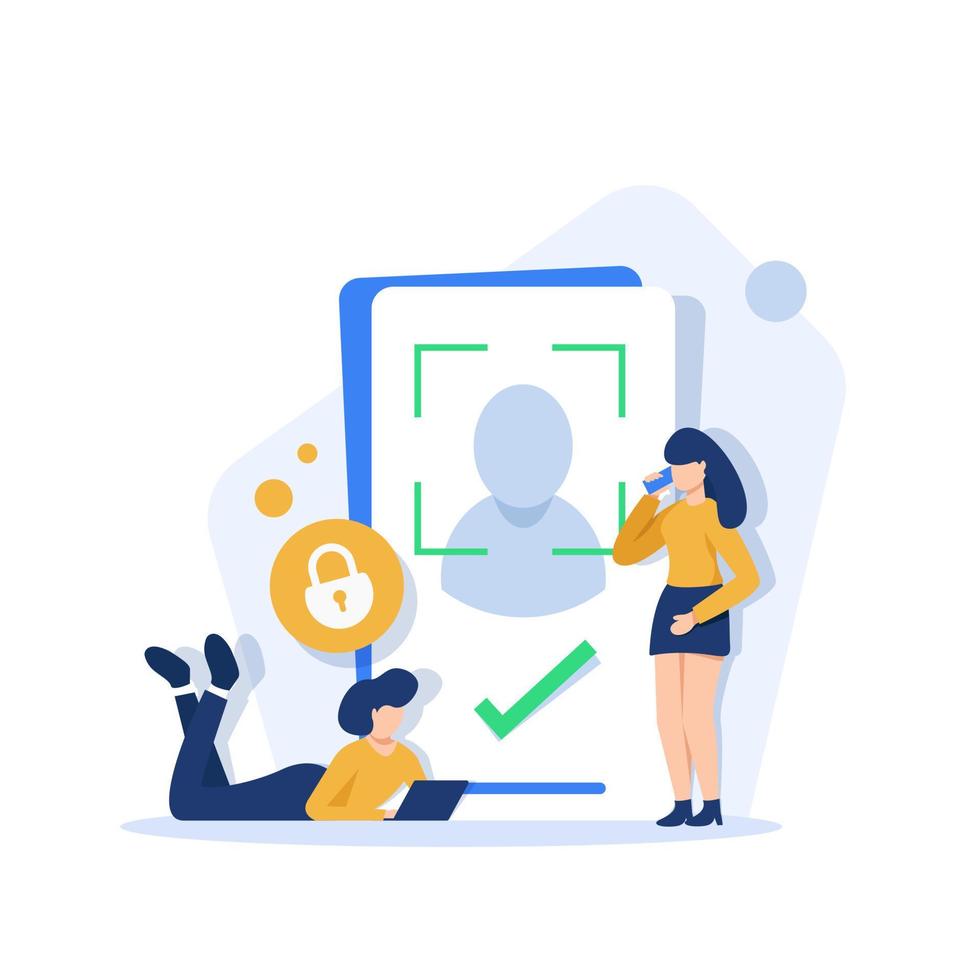The image is a digital illustration featuring two faceless female silhouettes, one lying on the ground working on a laptop and the other standing and talking on a cell phone. Both figures are wearing yellow shirts and blue bottoms, with the one lying down in pants and the one standing in a skirt. The primary colors used in the illustration are yellow, white, grey, and green. 

In the background, there are two large card-like signs. The card in the background is blue, while the one in the foreground displays a symbol for the torso of a human surrounded by green lines, along with a green checkmark and a yellow circle featuring a padlock. Above the figure lying on the ground, there's also a closed padlock symbol. The illustration has a minimalist style and could be part of an informational or instructional material, possibly related to security software or systems for telephones.